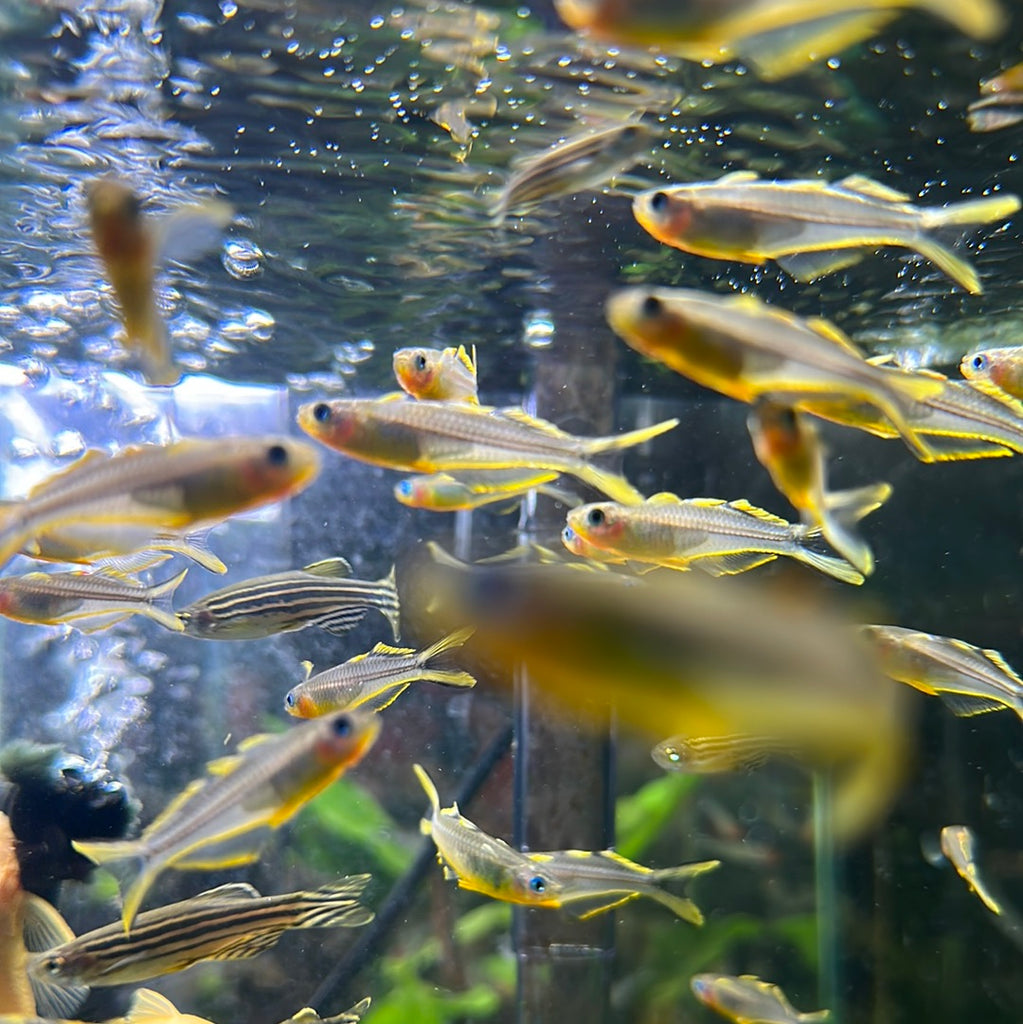This close-up image of an aquarium showcases a bustling aquatic environment teeming with approximately 20 fish, primarily concentrated near the surface. Most of the fish are slender, semi-translucent, and light gray, with bright yellow fins and hints of orange around their heads. A second, distinct species features bold black and white stripes, reminiscent of zebra patterns, with the same striking yellow fins and a touch of orange at the front. The fish swim in diverse directions, creating a dynamic scene with most moving left, while others swim diagonally or to the right. The tank's top surface is alive with bubbling water, disturbed by waves, and light shines into the tank from the left. At the bottom center, vibrant green plants and a scattering of sticks provide a naturalistic background, enhancing the tank's lively underwater ecosystem.